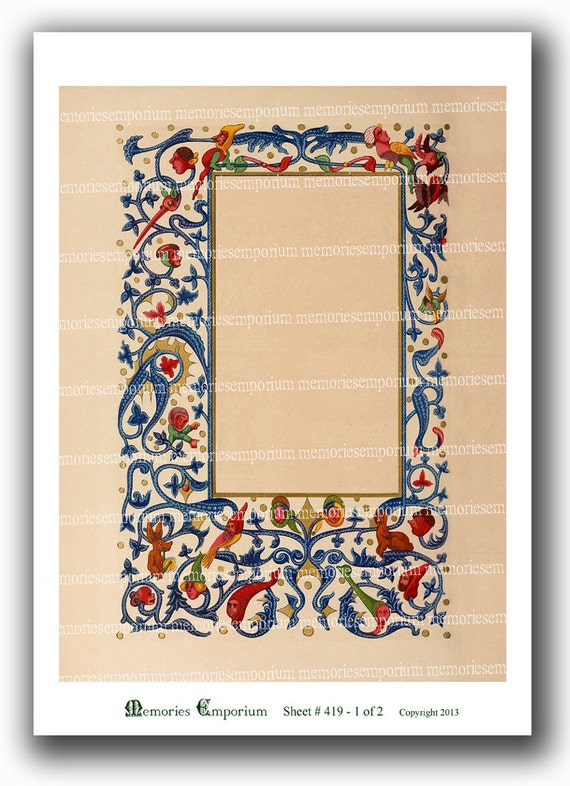The image depicts a digitally rendered, illuminated manuscript-style artwork on a parchment-like beige background. Dominating the center is an empty rectangular frame designed to hold a picture or serve as an initial letter in a medieval manuscript. This frame is richly adorned with intricate, swirling filigree that intertwines with various colorful elements, including small gnome-like faces, birds, demons, and animals such as rabbits. The illustration exudes a medieval aesthetic and Middle Eastern influence, marked by its vibrant, detailed imagery of plants and possibly fruit. At the bottom of the artwork, there is white text that reads "Memories Emporium, sheet number 419, one of two, copyright 2013."